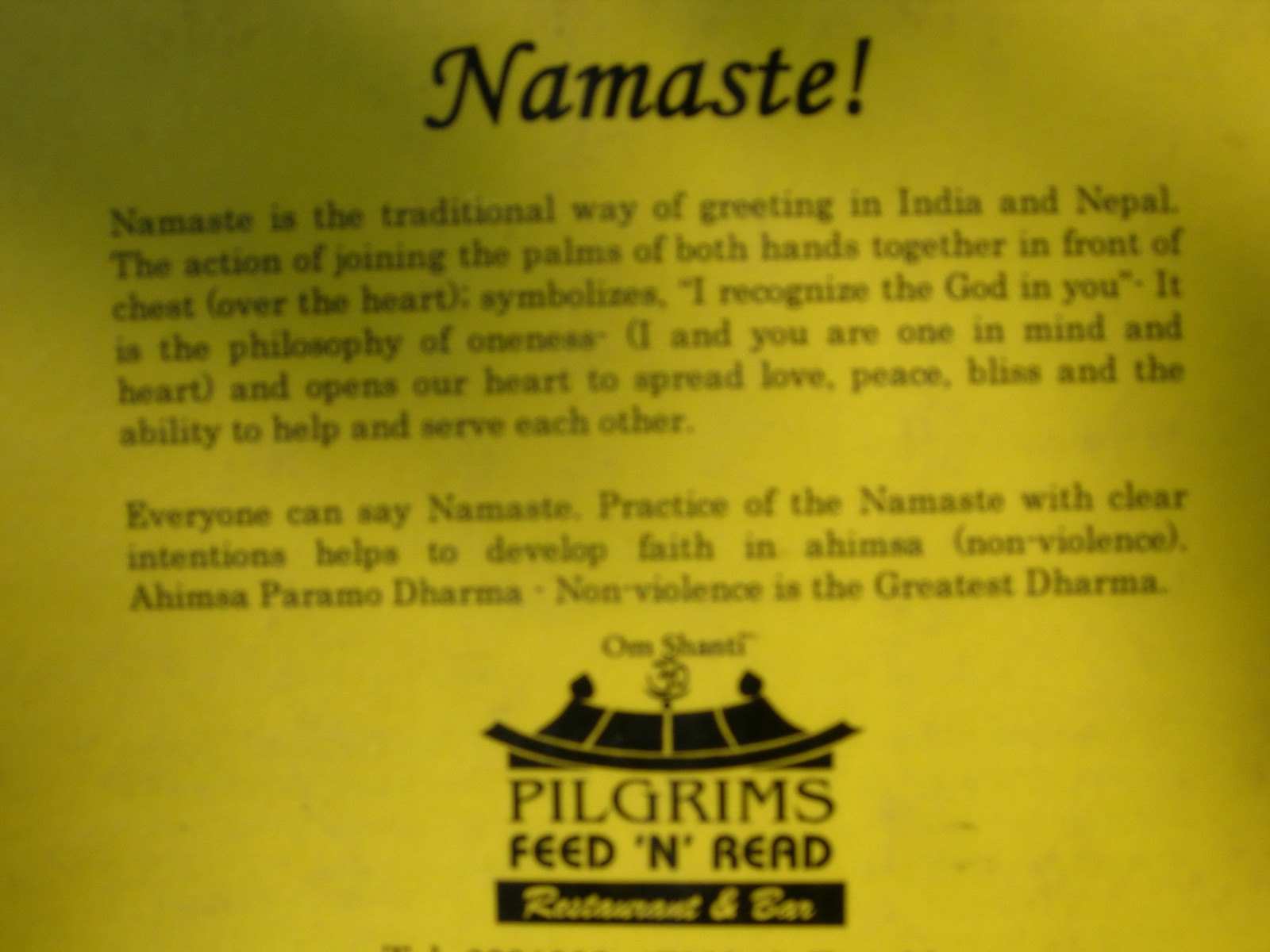In the image, there is a vibrant yellow card with prominent black text. At the top, in large black letters, it says "Namaste!" Below that, there is an informative description: "Namaste is the traditional way of greeting in India and Nepal. The action of joining the palms of both hands together in front of the chest symbolizes 'I recognize the God in you.' It embodies the philosophy of oneness, implying 'I and you are one in mind and heart,' and aims to spread love, peace, bliss, and the ability to help and serve each other. Everyone can say Namaste; practicing it with clear intentions helps develop faith and nonviolence, which is considered the greatest Dharma." Towards the bottom of the card, there is a simple black cartoon-style logo resembling a house roof, accompanied by the text "Pilgrims Feed and Read Restaurant and Bar."